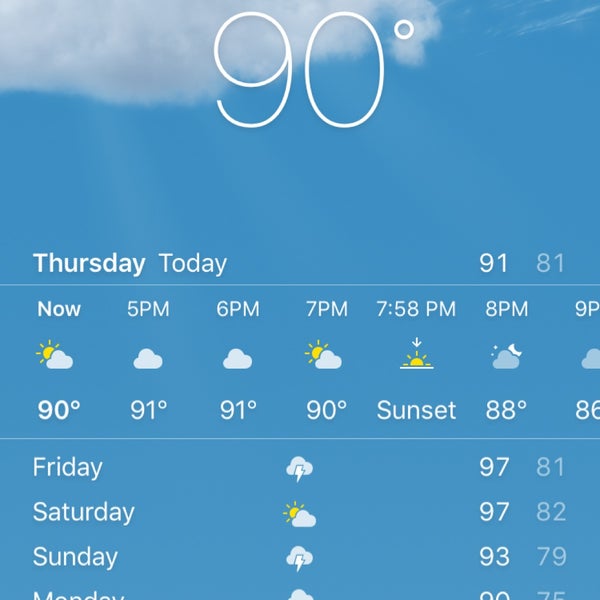The image depicts a weather forecast screen displayed on a cellphone, framed with a highly detailed layout. The backdrop showcases a stunning blue sky, interrupted only by a single, delicate cloud in the upper left-hand corner. Central to the image is the current temperature, prominently displayed as 90 degrees. The forecast for the day is presented below, with "Thursday" and "Today" inscribed above temperature details that indicate a high of 91 degrees and a low of 81 degrees.

Further down, the forecast is broken down by the hour:
- **Now:** Partly cloudy, 90 degrees
- **5 PM:** Fully cloudy, 91 degrees
- **6 PM:** Fully cloudy, 91 degrees
- **7 PM:** Partly cloudy, 90 degrees
- **7:58 PM:** Sunset
- **8 PM:** 88 degrees with the moon peeking out from behind clouds
- **9 PM:** Partially visible, 86 degrees

Scrolling down to the bottom, a subtle gray line demarcates the extended forecast:
- **Friday:** Thunderstorms, high of 97 degrees, low of 81 degrees
- **Saturday:** Partly cloudy, high of 97 degrees, low of 82 degrees
- **Sunday:** Storms, high of 93 degrees, low of 75 degrees

The details for Monday remain incomplete, cut off at the bottom edge of the display.